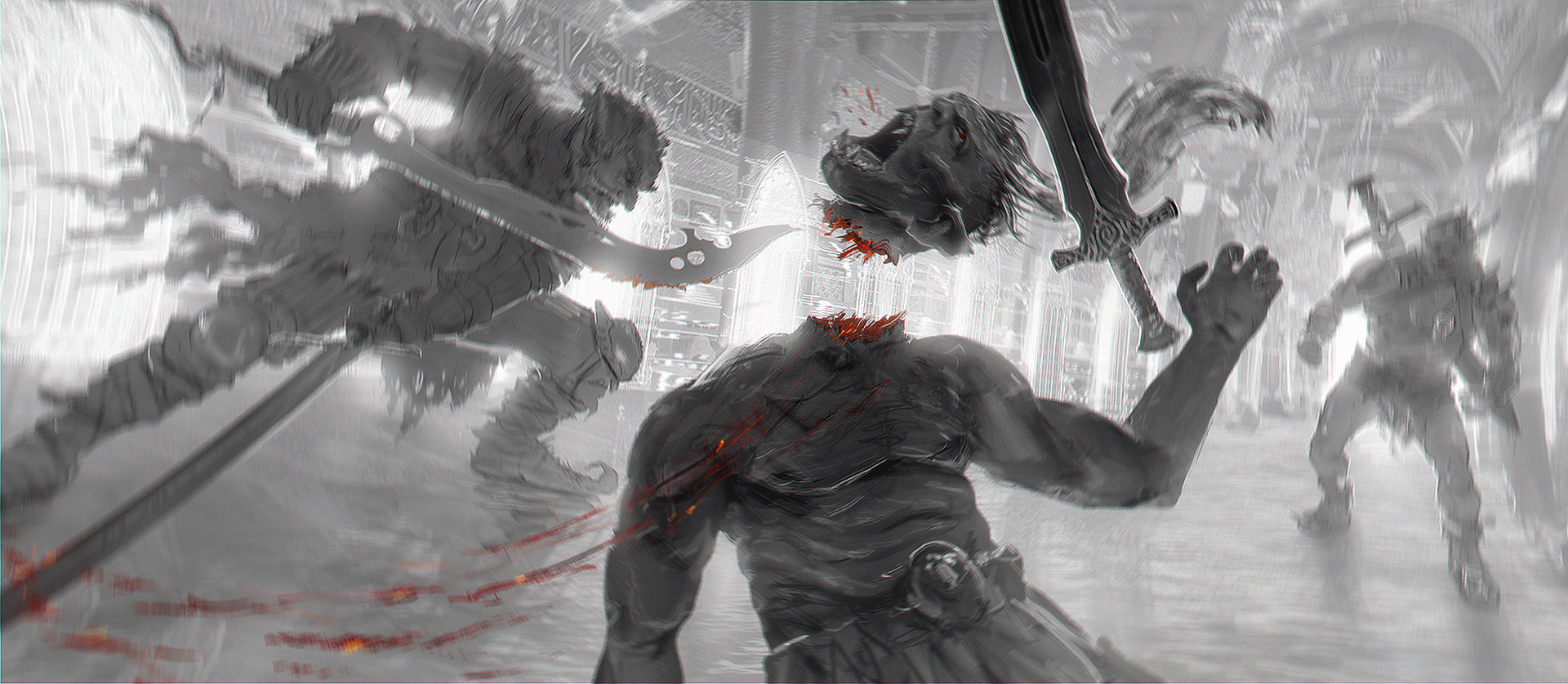The image is a highly detailed black and white sketch, possibly computer-generated due to its high level of complexity. It depicts a brutal battle scene within a large, Gothic hall filled with curves, peaks, and high ceilings. The primary focus is on three grotesque, monstrous warriors reminiscent of the orcs from 'The Lord of the Rings.' 

At the front and center, one warrior has just been decapitated. His severed head, with long flowing hair and an expression of rage, is mid-air, facing upwards with blood gushing from his open mouth. The body, now headless, has a gory, blood-splattered neck and an outstretched hand, bent at the elbow, with the sword no longer grasped. Blood splatters form a semicircle pattern around the fallen figure, emphasizing the violence of the scene.

Above this figure, another creature, with an angry face and mummy-like wrapping, is charging forward with a sword in hand. Further in the background, another warrior stands with a large sphere strapped to his back and a sword secured in a clasp. This figure appears ready to engage, adding to the intensity of the conflict. The entire scene, rendered in shades of black and gray, is dominated by the gothic architecture and the sheer brutality of the moment.